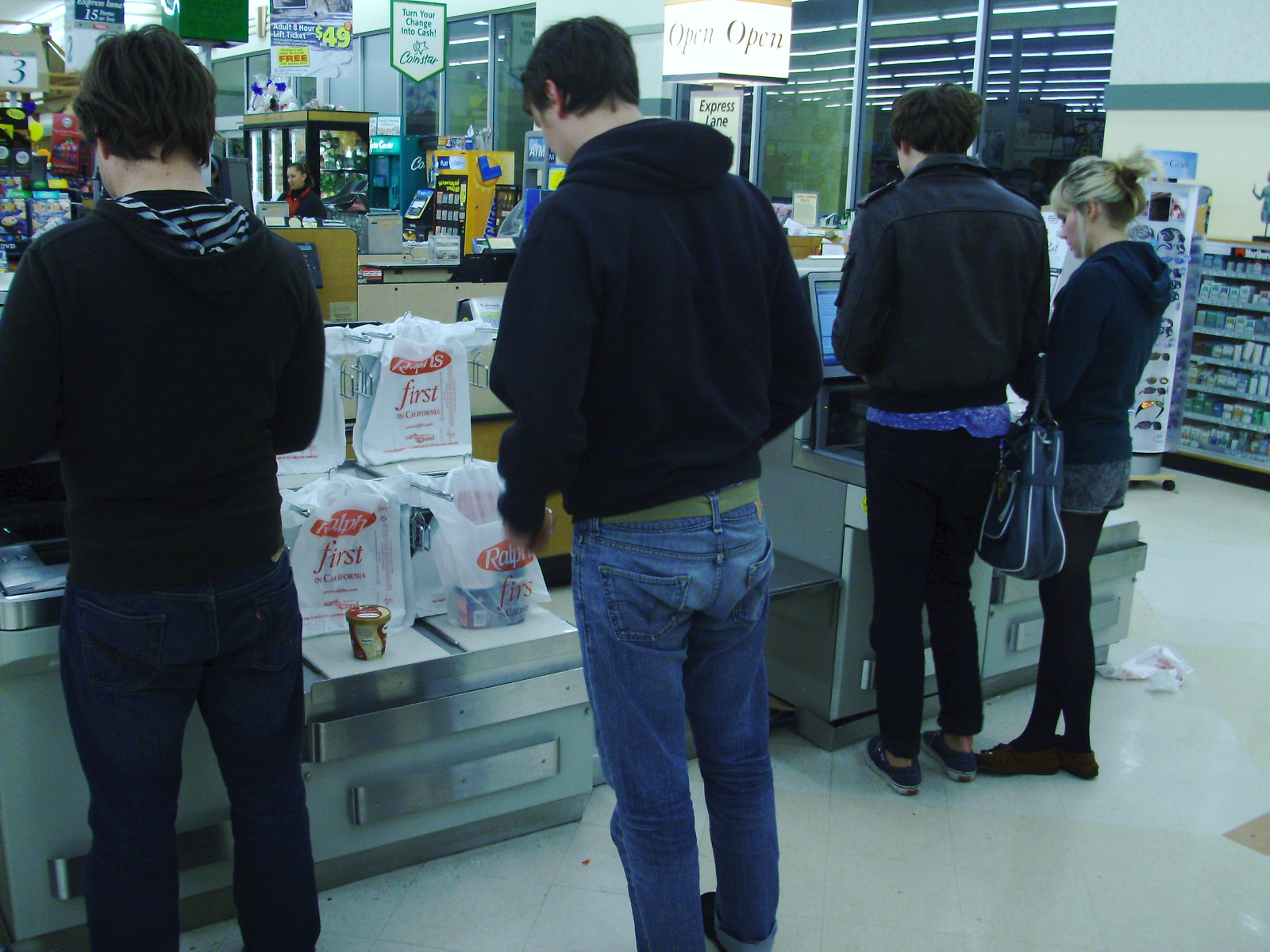In this detailed image of a bustling Ralph's grocery store at nighttime, we observe four individuals engaged in various stages of self-checkout. Two women, dressed in black with their hair pulled back into ponytails, stand at a checkout station. One woman, shorter with blonde hair, and the other, with darker hair, are focused intently on scanning their items. Nearby, a man waits as another man completes his purchase, standing near the white grocery bags marked with red lettering that blur the word "First." 

The scene is colorful and dynamic, with several checkout stations visible, each occupied by young shoppers. There's a shopper who appears to be buying and bagging ice cream. Brightly colored signs hang from the ceiling, one of which reads "Express Lane Open," amidst various price listings. In the background, an employee moves about, and a lottery ticket machine stands ready for players. The large, opaque windows reveal the night outside, hinting at the late-hour energy within the store.